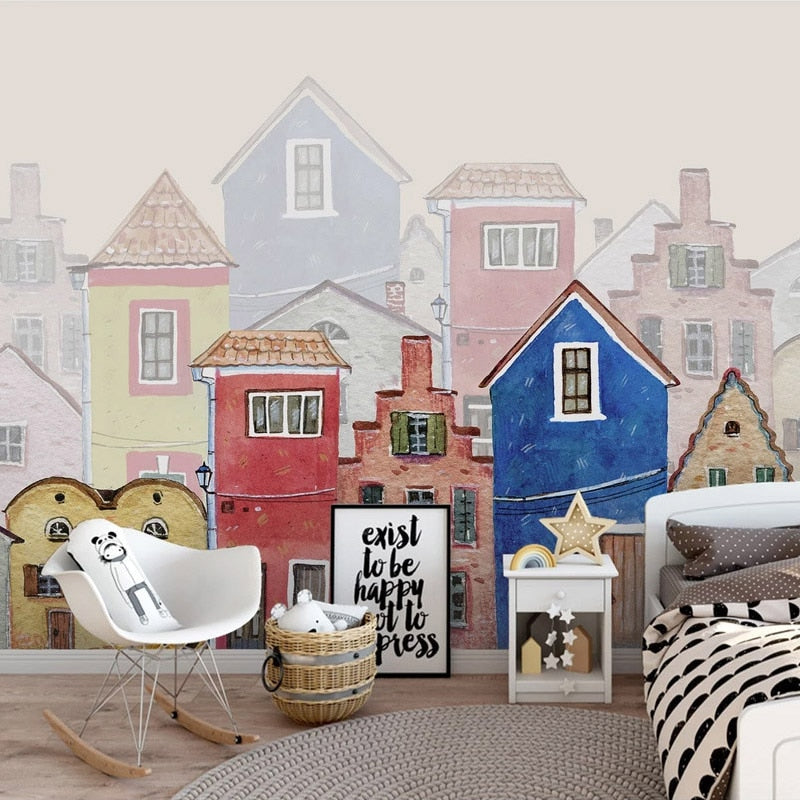This image depicts a charming, whimsical kid's bedroom featuring a detailed mural of a quaint European city with multi-colored old buildings—some blue, red, and yellow—receding into the distance where the colors become more muted. On the right side of the room, there is a child's bed with a white headboard and baseboard. The bed is adorned with a black and white quilt, and gray pillows and mattress covers with white polka dots. To the left of the bed stands a white wooden nightstand decorated with star motifs and a small rainbow trinket. A black and white framed sign leans against the wall, reading, "Exist to be happy, not to impress," though part of the text is obscured. Below, the floor is light brown wood, complemented by a beige circular rug with a concentric pattern. In front of the mural, a white rocking chair with wooden rockers holds a plush toy resembling a girl in a panda hat. Adjacent to the chair is a wicker basket with black handles, containing a few pillows. This meticulously designed room beautifully blends playful elements with comforting decor, making it a perfect sanctuary for a child.